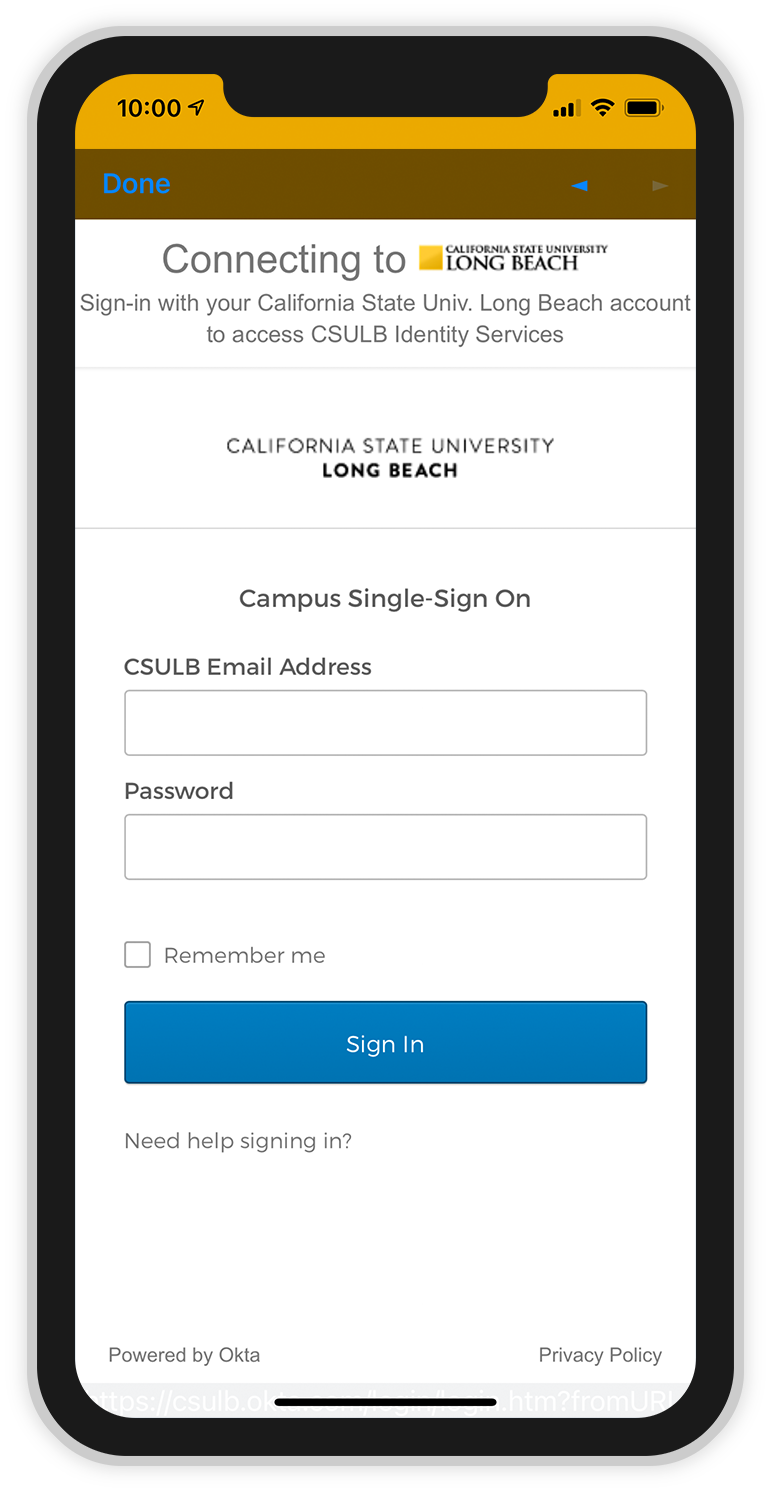The image showcases a mock-up of a phone app, framed by the outline of a newer iPhone. The top-right corner indicates that it is either 10 a.m. or 10 p.m., and displays the location symbol, three signal bars, and full Wi-Fi strength. The phone's battery appears nearly full.

Central to the image is a login screen for California State University Long Beach (CSULB). The webpage prompts users to "Sign in with your California State University Long Beach account to access the CSULB Identity Services." The school's name and the phrase "Campus Single Sign-On" also appear prominently.

In the upper left corner, there's a blue-text "Done" button. Below the sign-in instructions, there are fields for the user's CSULB email address and password. An unchecked box labeled "Remember me" appears below the password field, alongside a blue "Sign In" button. Additional text at the bottom offers assistance with "Need help signing in," and mentions that the service is "Powered by Okta," followed by a link to the private policy and the webpage’s URL.

The background of the login webpage is predominantly white, but the overall backdrop of the screen has a yellow tint, providing a subtle contrast.